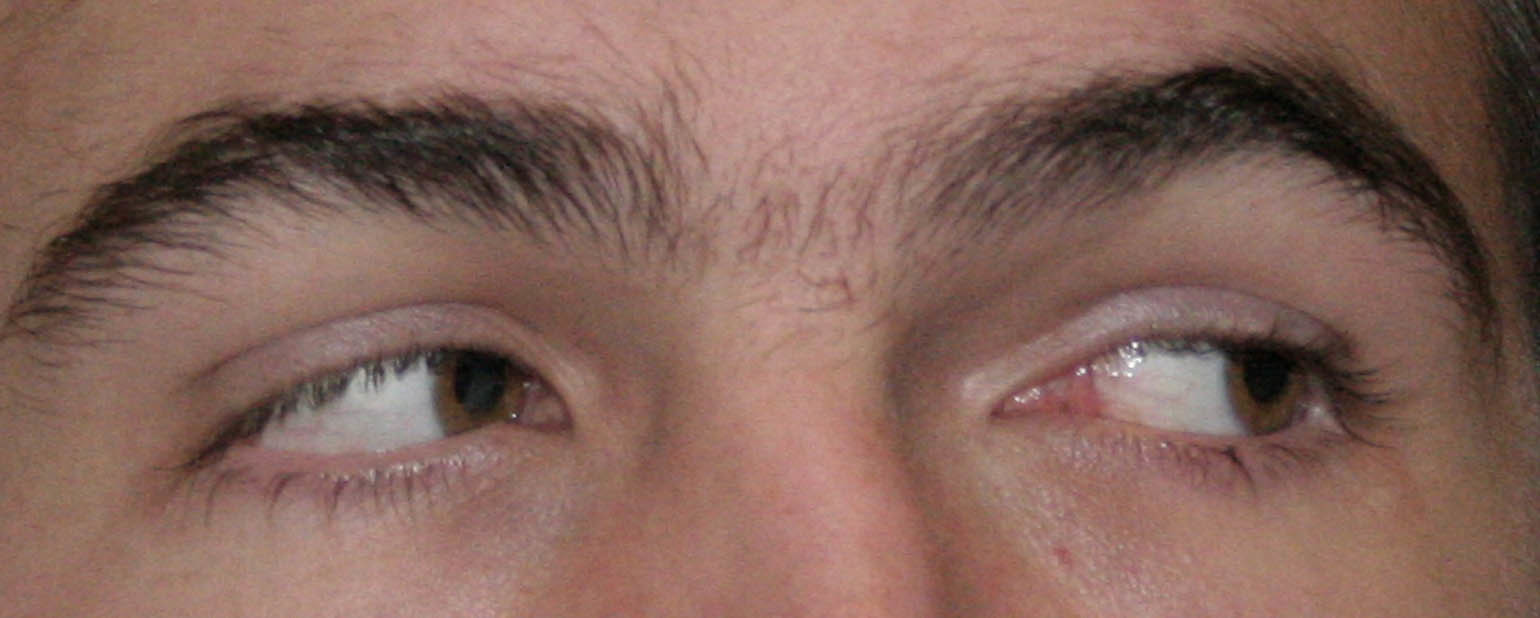This landscape-oriented, color photograph captures a close-up of a man's eyes and eyebrows in a narrow horizontal frame. The man, who has light brown eyes and thick, dark eyebrows that nearly form a unibrow, is gazing toward the left side of the image with an expression that conveys suspicion and worry. His eyes are framed by dark eyelashes on both the upper and lower lids. Only the upper section of his face is visible, extending from just above his eyebrows to midway down his nose, with some eyebrow hairs on the bridge of his nose. The skin around his eyes looks healthy, without any dark circles, and the setting maintains a realistic, photo-representational style.